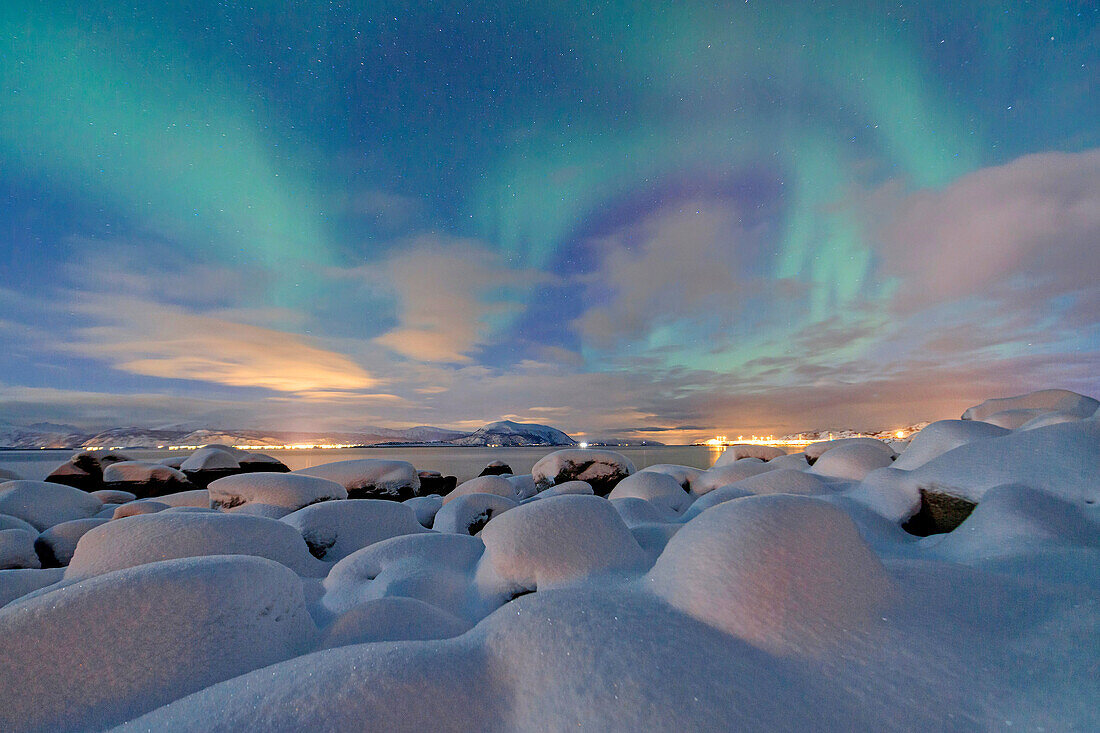The image depicts a serene, snowy landscape with a thick, smooth, and powdery layer of untouched snow covering mounds and rocks in the foreground. The snow appears natural and undisturbed, creating a peaceful scene. Past the snow, a body of water stretches across the image, leading to a distant mountain visible straight ahead. On both sides of the mountain, the lights of a town twinkle against the horizon. The sky is a captivating blend of colors, featuring shades of bright blue, aqua, and hints of purple. It also has areas where golden light from the sun illuminates parts of the clouds, adding warmth to the scene. Some white clouds scatter across the sky, with the sunlight peeking through and casting a subtle glow. There are also green highlights in the sky, contributing to the image's overall beauty. The combination of the tranquil snow-covered rocks, the colorful and dynamic sky, and the distant town lights creates a picturesque and calming winter scene.